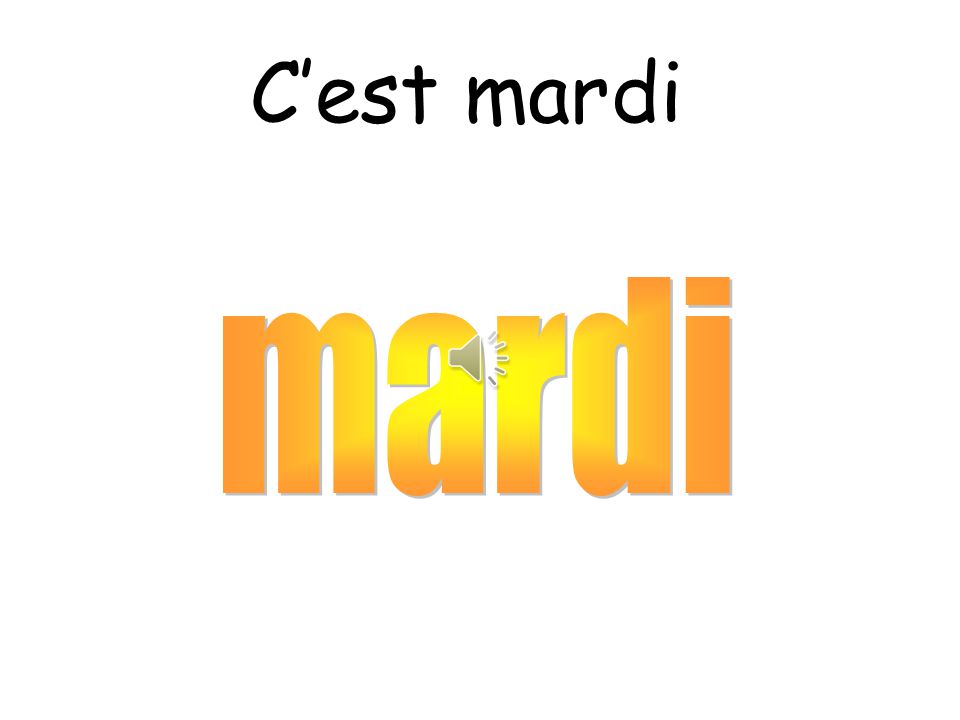The image features a white background with two lines of text in distinct styles. At the top, there is black text in Comic Sans that says "C'est mardi," with all letters in lowercase except the initial "C." Below this, in the center of the image, is the word "mardi" again, but in a large, bold, and colorful font. The letters of "mardi" are orange with a gradient that transitions to bright yellow towards the center. Additionally, embedded in the middle of the "a" or near the top right of the "a" in this colorful "mardi," there is a small gray speaker icon, like a volume icon seen on computers or phones.